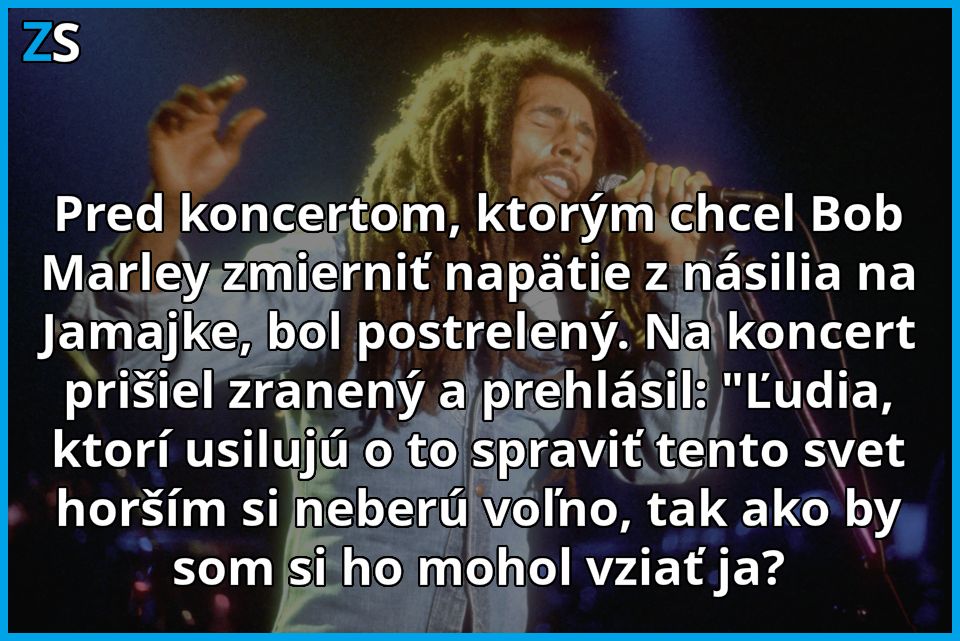The image depicts Bob Marley, the renowned singer who passed away in the 1980s, captured in an evocative concert scene. Bob Marley, a black man with distinctive black dreadlocks and a black goatee, is deeply engaged in his performance, closing his eyes and singing passionately into a black microphone with a silver spherical head, which he holds with his left hand. His right arm is extended into the air, adding to the intensity of the moment. Clad in a light blue button-up long-sleeve shirt, he stands out against the vivid blue and dark-toned background.

The photograph is bordered with a light blue frame, and in the upper left corner, there are the initials 'Z' and 'S'—the 'Z' in blue with a black outline and the 'S' in white with a black outline. Superimposed over the image is a substantial amount of white text with a black border, center justified and written in what appears to be a Slavic or Eastern European language, comprising seven lines. This text likely discusses Bob Marley's life and career. The lower part of the image features lights that could represent crowd members or bandmates, adding to the concert ambiance.